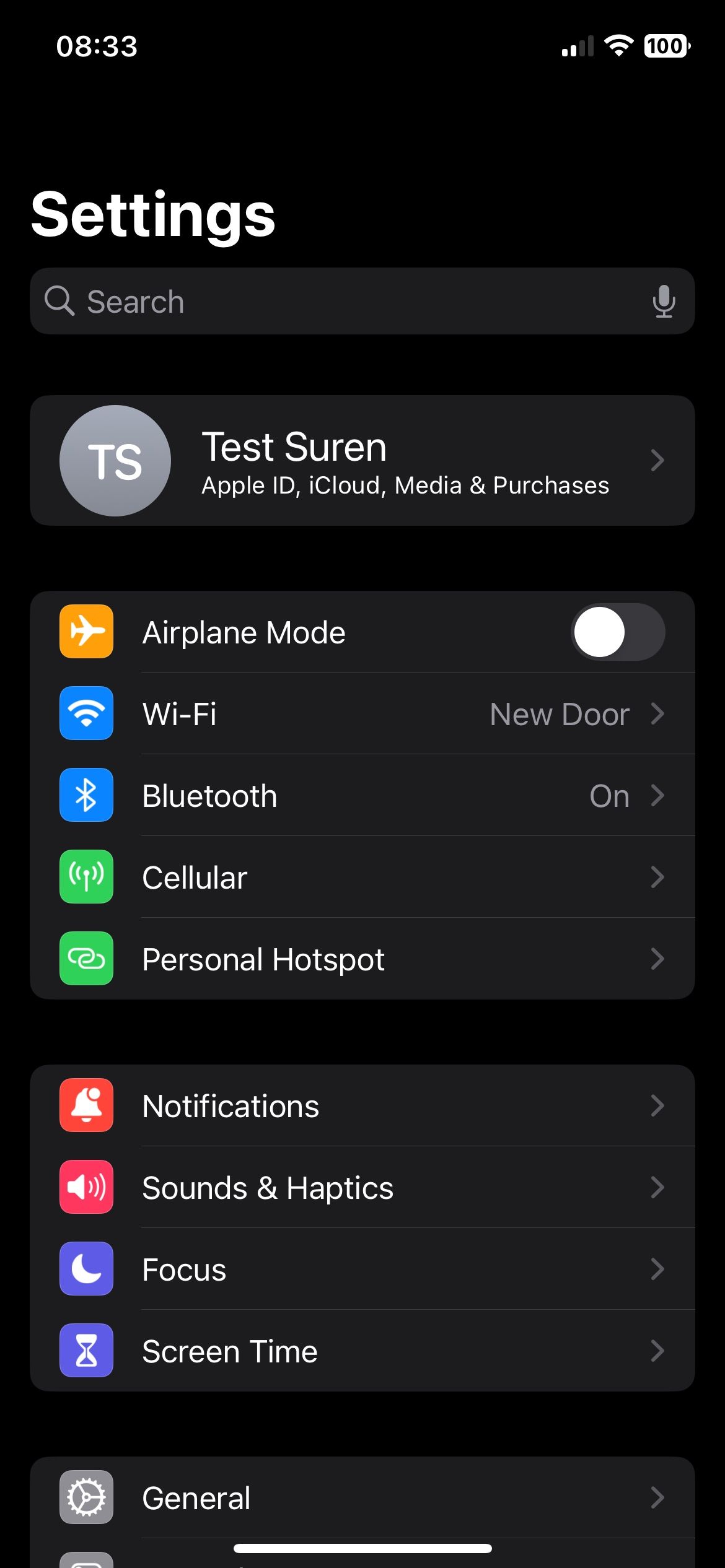The image is a screenshot of a smartphone displaying the "Settings" menu. At the top, the word "Settings" is prominently featured in bold white text. Beneath this heading is an oval search bar containing a magnifying glass icon and the text "Search," along with a microphone icon on the right-hand side.

Immediately below the search bar, there is a black space followed by a gray circle with the initials "TS" inside it. To the right of this circle, the text reads "Test Surrender," and beneath this, it indicates "Apple ID, iCloud, Media & Purchases" with a right-pointing arrow next to it.

Further down, another black space separates the previous section from a series of settings options, each accompanied by their respective icons on the left:
1. **Airplane Mode:** Depicted with an airplane icon and an off-toggle switch on the right.
2. **Wi-Fi:** Shown with a Wi-Fi signal icon and the text "New Door," followed by a right-pointing arrow.
3. **Bluetooth:** Illustrated by a Bluetooth icon, with "Bluetooth" written to its right, and another right-pointing arrow.

The menu continues with more options such as:
- **Cellular:** Indicated by a green cellular icon.
- **Personal Hotspot**
- **Notifications**
- **Sounds & Haptics**
- **Focus**
- **Screen Time**
- **General**

Each of these additional options features corresponding icons.